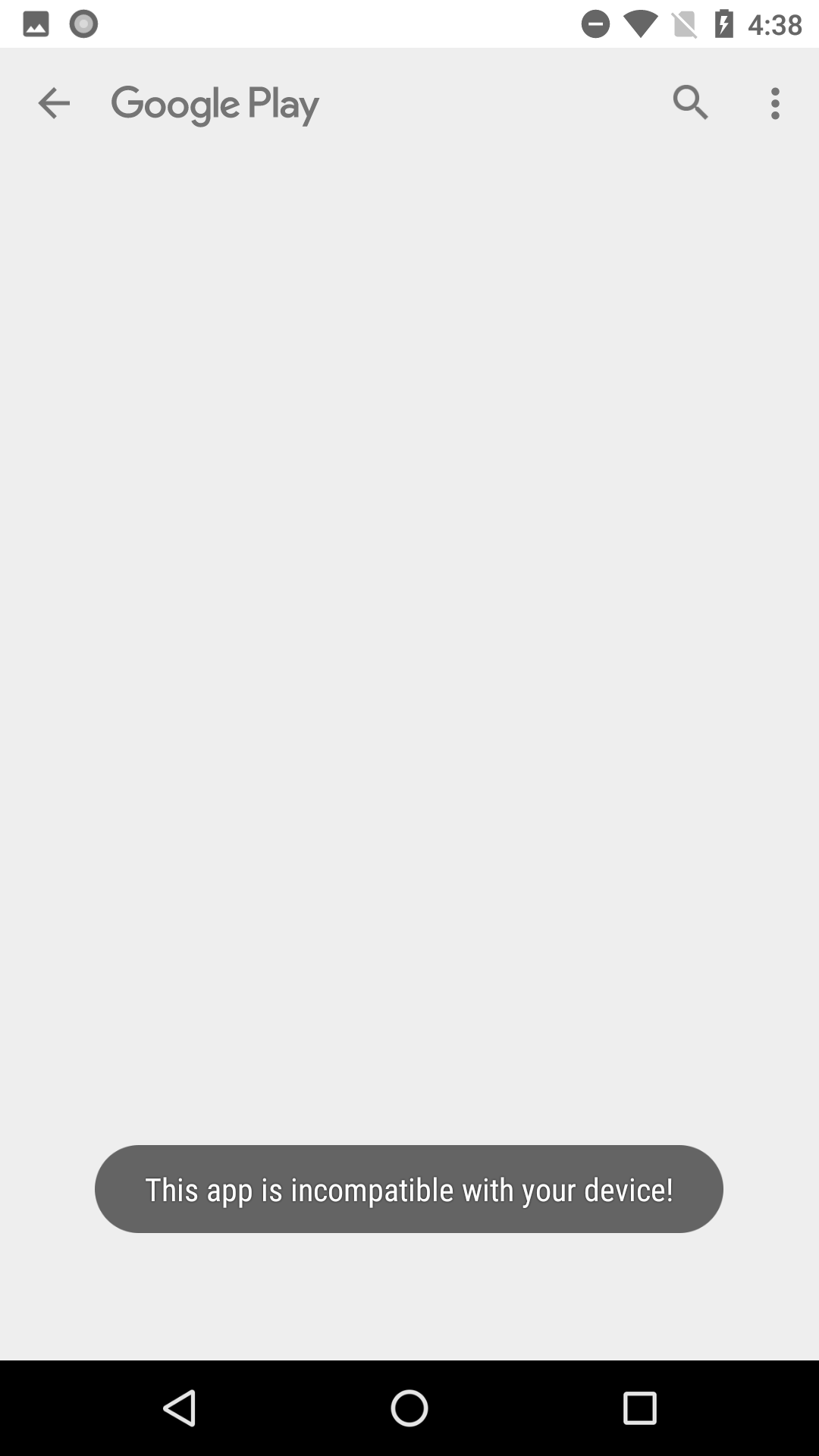In the image, a person attempts to access Google Play on their smartphone, but the app is unresponsive, indicating that it is incompatible with the device. The screen displays a disclaimer in gray at the bottom, notifying the user of this incompatibility. There is no visible app icon, reinforcing the app's unavailability. 

The smartphone's black taskbar is shown at the bottom, featuring a left-pointing arrow resembling a triangle, a circle, and a square. At the top left corner, there's an icon of a black box with a mountainscape and a double circle beside it. The time on the device reads 4:38, and a battery icon with a lightning bolt signifies that the battery is currently charging. Additional icons include a funnel symbolizing Wi-Fi and a circle with a minus sign. The text "Google Play" appears grayed out underneath the left icon, followed by a left arrow, and on the far right, there is a magnifying glass next to three vertical dots. 

The grayscale display reinforces the app's inaccessibility, with the majority of the elements rendered in gray, except for the top taskbar and the icons, which stand out in gray, and the bottom bar that is black with white shapes.